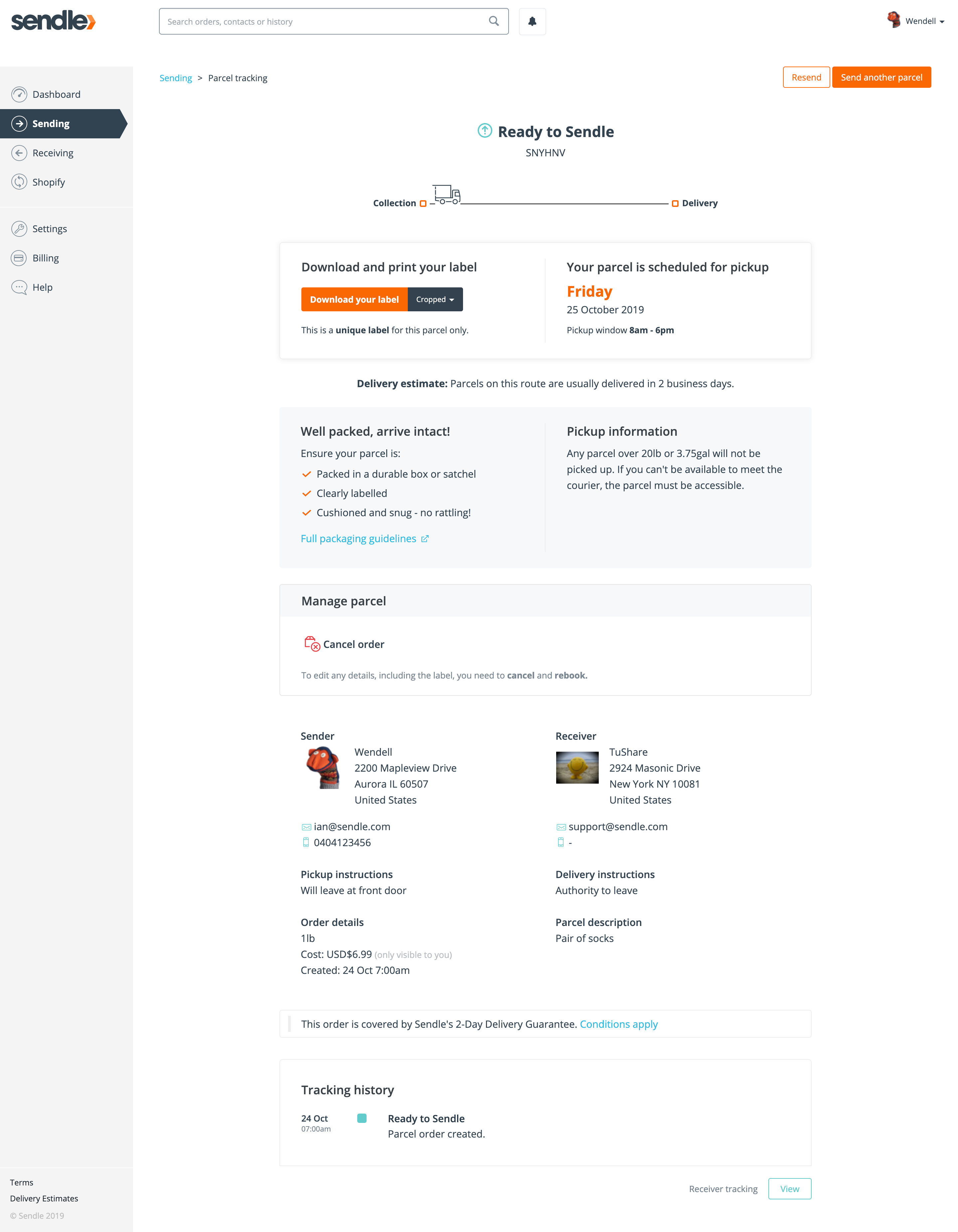This is a detailed image of a Sendle (spelled S-E-N-D-L-E) website interface.

The website branding prominently features the company name "Sendle" in blue, with an orange arrow positioned close to the letter "E". At the top of the interface, there is a space bar and two colored bars—a longer orange bar next to a white bar outlined in orange. Additionally, an icon accompanied by a word in black appears at the top.

On the left-hand side, various menu items are listed, with "Sending" highlighted in black. Dominating the center of the page is a message that reads "Ready to Sendle," placed beside a blue plus sign.

Below this, a graphical representation of a truck is displayed, suggesting motion towards the right. Further down, an orange download button invites users to "Download and print your label." An important notification in orange indicates that "Your parcel is scheduled for pickup Friday, October 25, 2018," along with details on the pickup time and delivery estimates.

The website provides extensive information about the delivery, including options to "Manage your package" and "Cancel your order." It features an image of a sender, illustrated as an orange character, and a receiver with a profile picture. Users are also given detailed pickup instructions and order details.

A specific note mentions that "This order is covered by Sendle's two-day delivery guarantee," followed by a tracking history section in blue, allowing users to track their package.